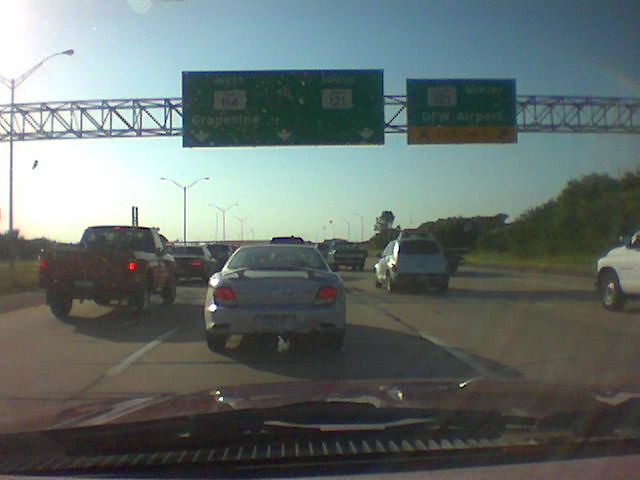This is a color photograph taken from inside a vehicle, looking through its windscreen on a busy freeway in North America, specifically in the Dallas-Fort Worth area. The scene is set either during sunrise or sunset, as indicated by the sun positioned to the left, casting a warm glow, and contrasting with the blue sky to the right. The freeway consists of at least five lanes, and we are positioned in the second lane from the left. There is a grass median to the left of us and another one farther to the right.

Above the lanes, green traffic signs hang from a steel gantry made of silver scaffold poles. These signs display typical freeway information with white lettering. The sign directly above us has three downward-pointing white arrows, with the left arrow indicating "Grapevine." The sign to the right identifies the DFW Airport, elucidating that DFW stands for Dallas-Fort Worth. Other highway indicators include mentions of highways 114 and 121.

Traffic is heavy, with numerous vehicles visible. Directly ahead is a white small sedan, to the immediate left is a red pickup truck with its brake lights on, and to the right is a silver SUV and a white truck in the far-right lane. The clarity and volume of vehicles suggest slow-moving traffic. Streetlight poles line the sides of the freeway, and the right side is bordered by bushes and trees.